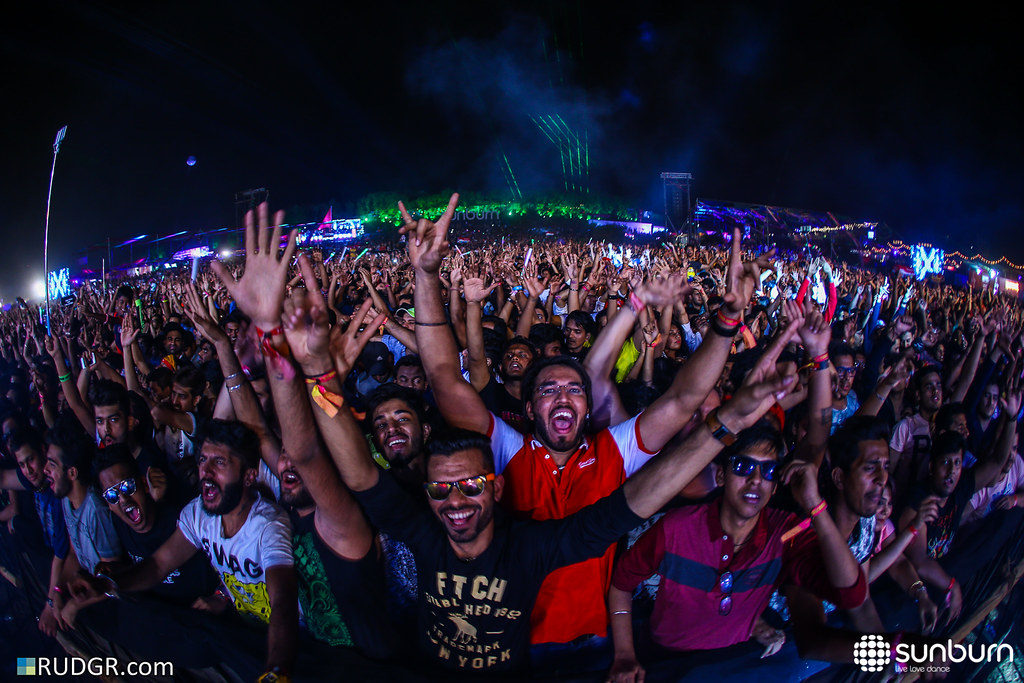This is a horizontally oriented, nighttime photograph capturing the joyous energy of a massive crowd, likely at a music festival. The image is filled with thousands of people, their hands raised in excitement, some with open palms and others with fingers pointed up. Wristbands, likely pink, mark the festival attendees who are dressed in colorful shirts. Neon glow sticks and the occasional pair of sunglasses add to the vibrant atmosphere. The crowd is a sea of smiling and cheering faces, with a diverse mix of men and women all reveling in the moment.

In the background, green lasers and an array of bright lights, including bluish-purple neon and large bulb lights, pierce through the smoky air, suggesting a spectacular stage performance or laser show. The backdrop features indistinct green figures and structures that add to the mystery and allure of the event. The photograph appears to be taken in a region with a darker complexion populace, possibly India or the Middle East, as inferred from the crowd's appearance.

At the bottom-left corner of the image, the text "rudgr.com" is visible, while the bottom-right corner displays the text "sunburn" accompanied by a round emblem, anchoring the festive scene with a sense of branding and location.